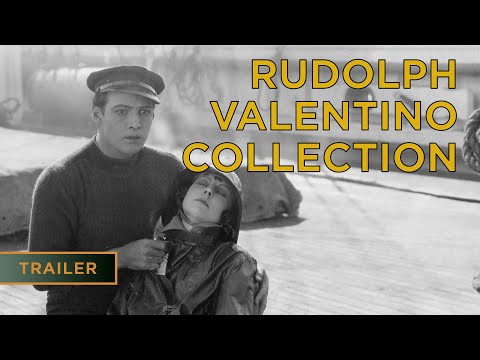This black and white, horizontal rectangular movie poster or trailer screenshot features a dramatic scene with two central characters—a man and a woman. The poster is bordered in black at the top and bottom, each border about an inch or two thick. In the image, a young man, appearing to be between 25 and 30 years old, wearing a long-sleeved turtleneck sweater and a hat or cap that resembles a policeman's cap or army beret, is holding a woman who looks to have fainted or passed out. The woman's eyes are closed, and she is dressed in a raincoat with a hood over her hair. She appears considerably shorter than the man and seems to be in a semi-upright position, supported by him. The man, who looks distressed and confused, is staring off into the distance with a hint of indignation. The background is heavily blurred, making it difficult to discern the exact setting, though it vaguely resembles a factory floor with brick ground. Yellow capital letters in the top right corner of the photo read "RUDOLPH VALENTINO COLLECTION," while the bottom left corner features the word "TRAILER" in orange or yellow capital letters with an orange border against the black banner.